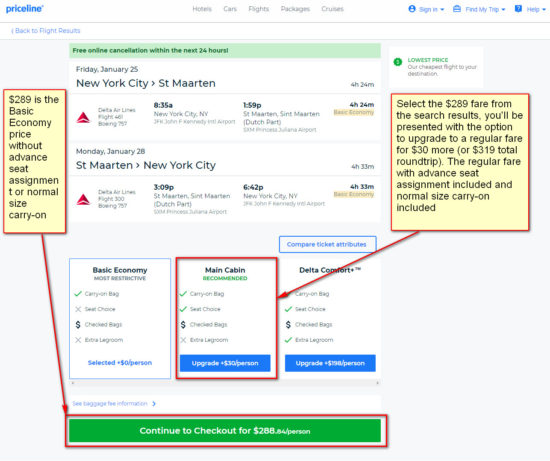**Caption:**

In the "Websites" screenshot, the top-left corner is labeled with the Priceline logo and a "Back to Flight Results" link. The same line also features navigation options: Home, Cars, Flights, Packages, Cruises, Sign In, Find My Trip, and Help. Below this, there's a notice offering free online cancellation within the next 24 hours, accompanied by an information icon indicating a lower price. Prominently displayed in a yellow box, the message reads: "$2.89 is the basic economy price without advanced seat assignment or normal-sized carry-on."

The flight details follow: 
- **Outbound**: Friday, January 25, from New York to St. Martin on Delta Air Flight 835, landing at 1:59 PM.
- **Return**: Monday, January 28, from St. Martin to New York, Delta departs at 3:09 PM and arrives at 6:42 PM.

Ticket options include Basic Economy, Main Cabin, and Delta Comfort, with Main Cabin presently selected. At the bottom, a green bar prompts users to "Continue to Checkout" for $2.88.